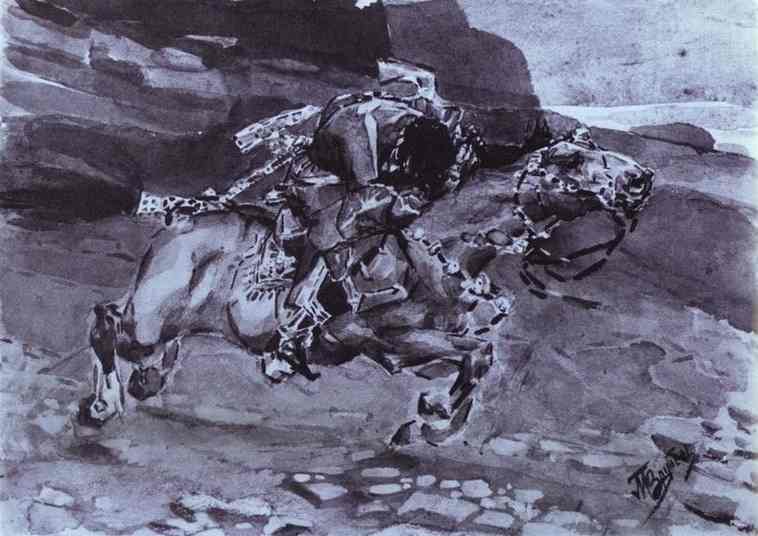This black, white, and gray drawing features a strong, galloping horse moving from left to right across a rocky, stony ground. The rider, hunched over with their head down, appears injured and leans forward on the horse, their feet resting in visible stirrups and something draped from their back down to the rear of the horse. Both the rider and horse exhibit a squared, blockish musculature style. The background showcases tall rock cliffs and sparse vegetation, with a gray sky and a dot representing the sun in the upper right corner. The lower right corner bears the artist's signature, which is somewhat indecipherable, potentially reading as J-M-B-A-Y-S-T-E-R or a variation thereof.